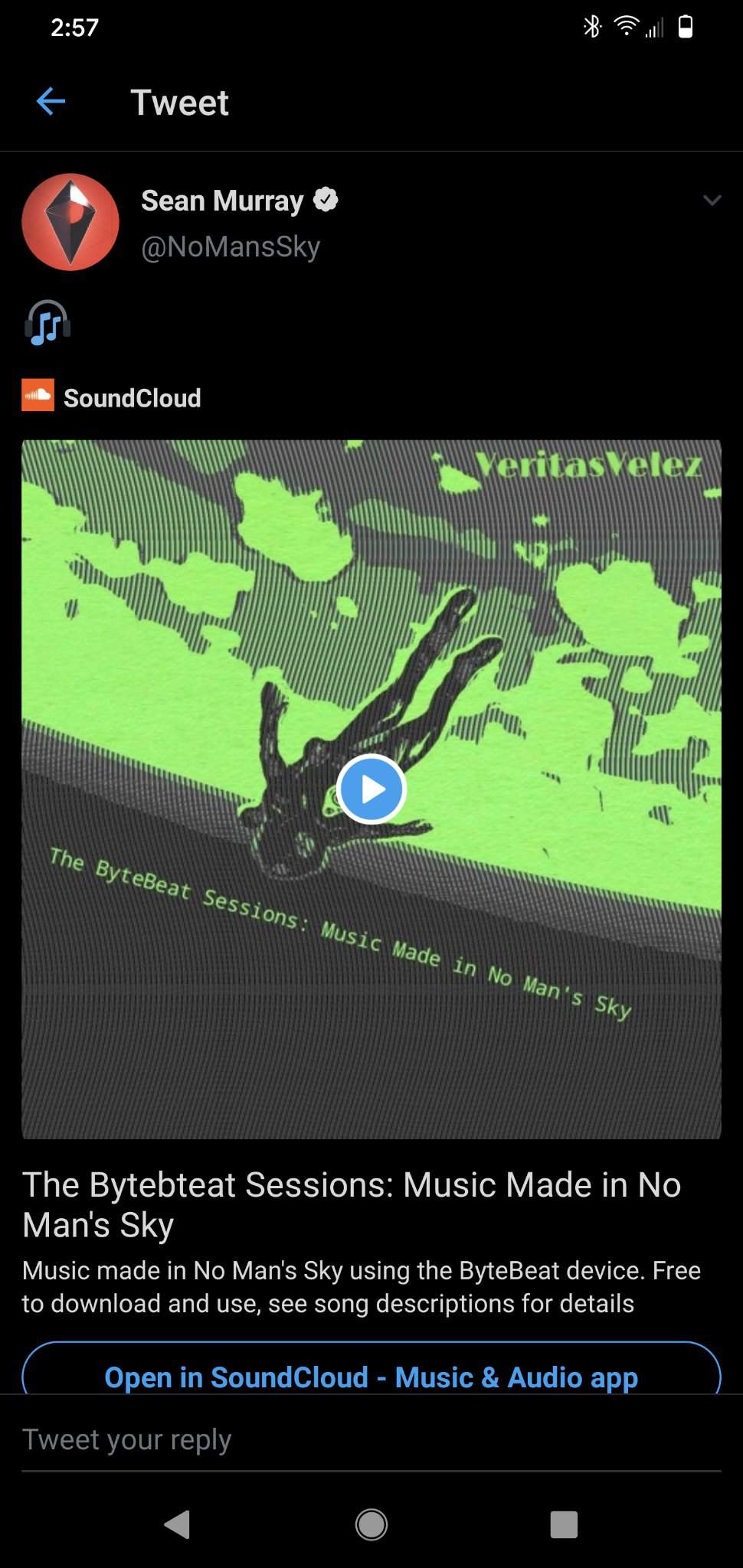**Image Description:**

The screenshot is from a cell phone display with a black background. The status bar at the top shows the time on the left, and icons for Bluetooth, Wi-Fi, cellular reception, and battery level on the right, all in white.

Just below, two lines down on the left, is a blue left-pointing arrow, with the word "Tweet" in white, spaced about eight characters to the right.

A few lines below that is a profile section featuring an icon: a red circle with a black diamond. To the right of the icon, the name "Sean Murray" is displayed in white, accompanied by a black checkmark inside a white circle, indicating verification. His Twitter handle is located below his name.

Lower on the left side, there is a gray-outlined circle containing two blue musical notes, which is the SoundCloud logo. To the right of this logo, "SoundCloud" is written. Below this is a video preview with a blue and white play button centered within. 

The video thumbnail shows an upside-down person against a green and gray background. At the top right of the thumbnail, "Veritas Vitezz" is written. Below the thumbnail, large white text reads "The ByteBeat Sessions: Music made in No Man's Sky." In smaller white text beneath that, it says, "Music made in No Man's Sky using the ByteBeat device. Free to download and use, see song descriptions for details."

At the bottom, a partial blue border of a button is visible, which reads in blue text: "Open in SoundCloud - Music & Audio App."